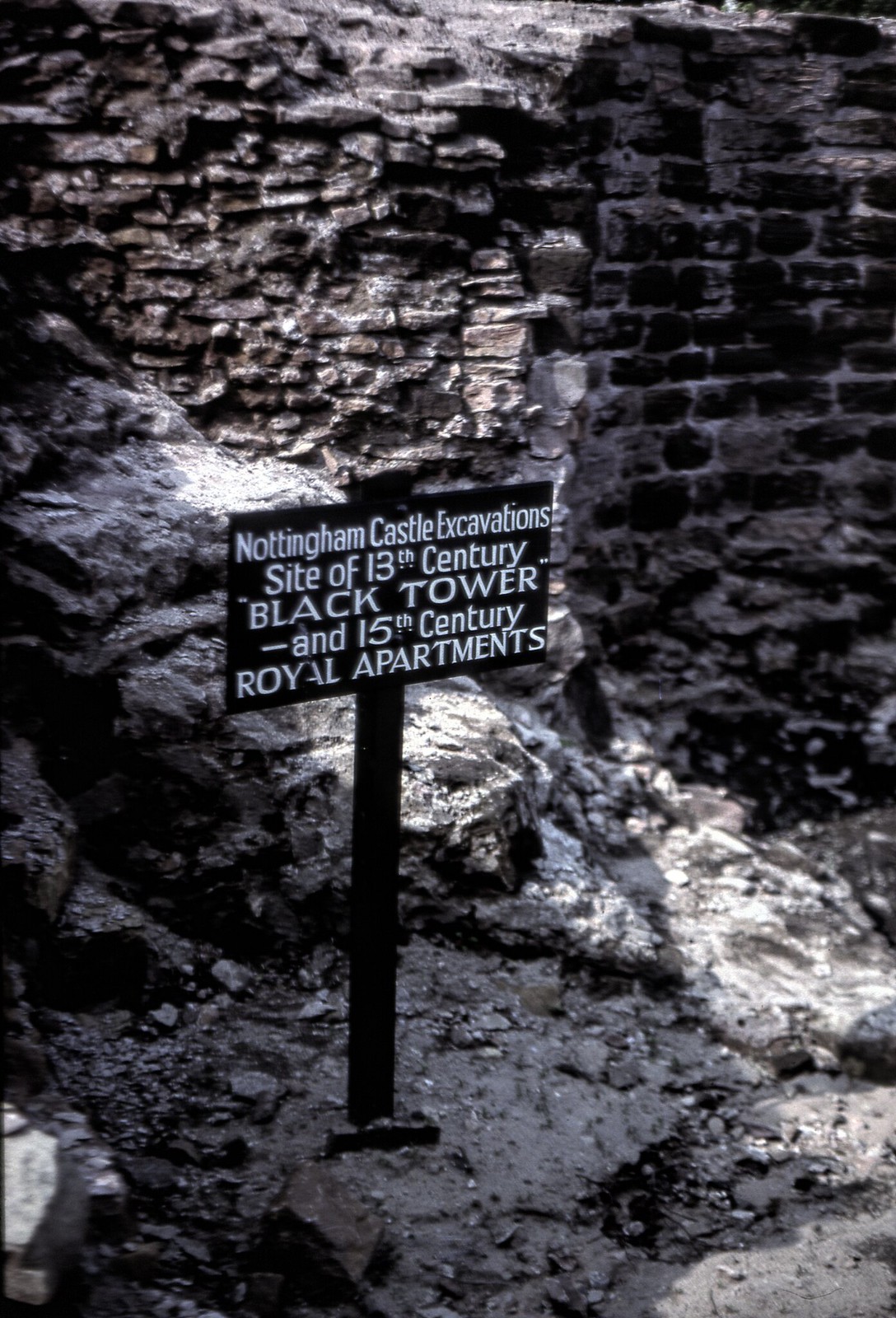The photograph depicts a stark, wintry scene featuring a deteriorating brick structure in the background, which could be remnants of a historical building possibly covered in remnants of snow. Prominently in the foreground, a black metal signpost juts out from a rocky, barren ground. The sign, with five lines of white text, reads "Nottingham Castle Excavations, Site of 13th Century Black Tower and 15th Century Royal Apartments," providing historical context about the site. The overall ambiance of the photo is notably dark, with the area shrouded in shadows despite the daylight. Dilapidated stairs and fragmented bricks are also visible, adding to the image's sense of decay and abandonment.